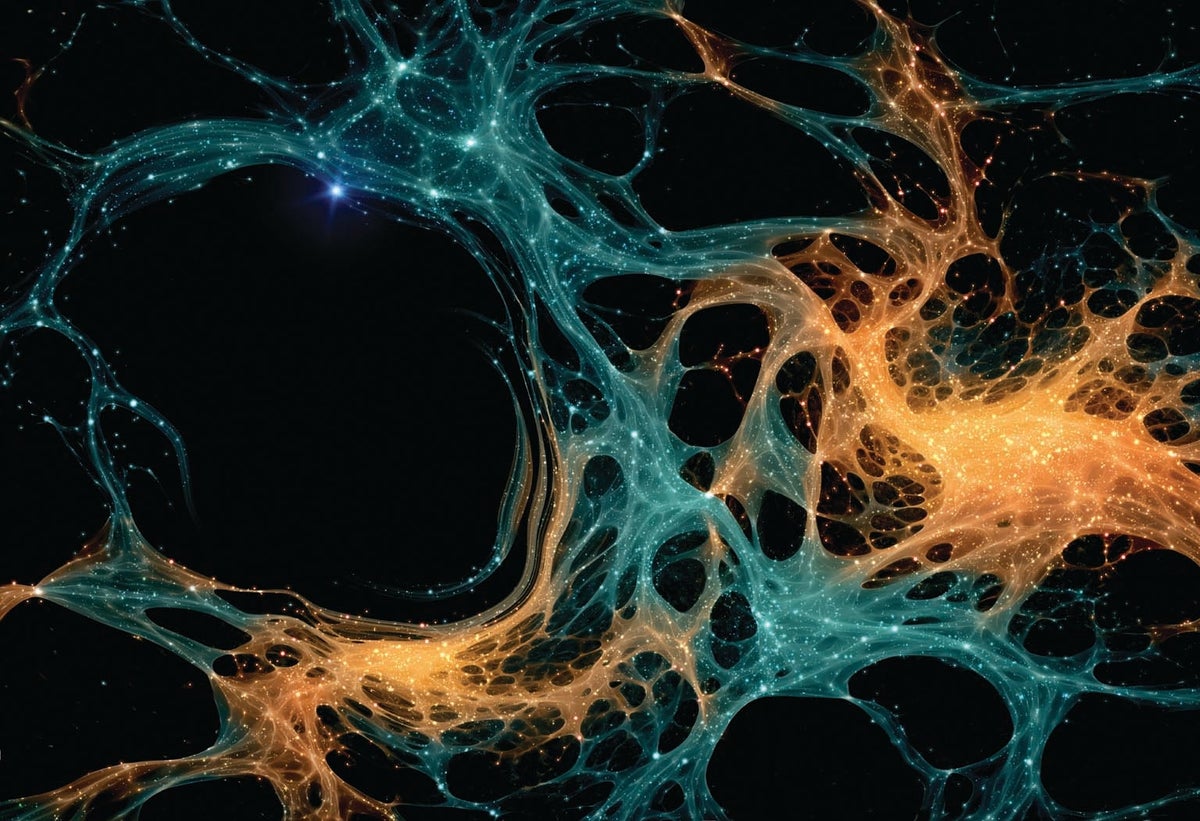The image features a completely black background adorned with abstract, tendril-like patterns resembling cosmic dust or a web-like dispersion of paint in water. The intricate structures appear semi-transparent, with a glowing, smoky quality. These patterns primarily consist of bright teal and subdued yet vibrant orange strands. The teal or bluish-green tendrils stretch diagonally from the top left corner to the bottom right, while the orange tendrils span from the right middle area toward the bottom left. The overall aesthetic evokes a desktop computer wallpaper or an abstract depiction of outer space, with glittery, cosmic elements that give the impression of stretched, glistening gold and silver threads interwoven throughout the dark expanse. The image is devoid of any text, allowing the viewer to fully immerse in its mesmerizing, otherworldly beauty.